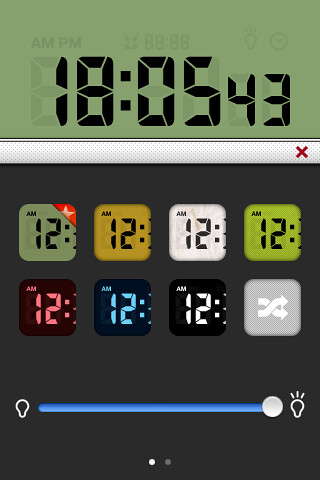The image displays a digital clock with various color schemes. At the top, a light green panel shows the date "1805-43" in digital text style, with "43" in a smaller font. A small red X appears at the top right of this panel. Below, numerous color options for the clock's display are presented against a dark gray background. These options include squares in yellow, white, different shades of green, pink, blue, and black, each showing the time "12:00 AM." The far right features a gray square with white crisscrossing arrows. At the bottom, a brightness adjustment section includes two light bulb icons: one empty and one with light rays emanating from it, indicating the ability to adjust the screen's brightness. The overall appearance suggests that the image is likely a screenshot from a smartphone settings menu.